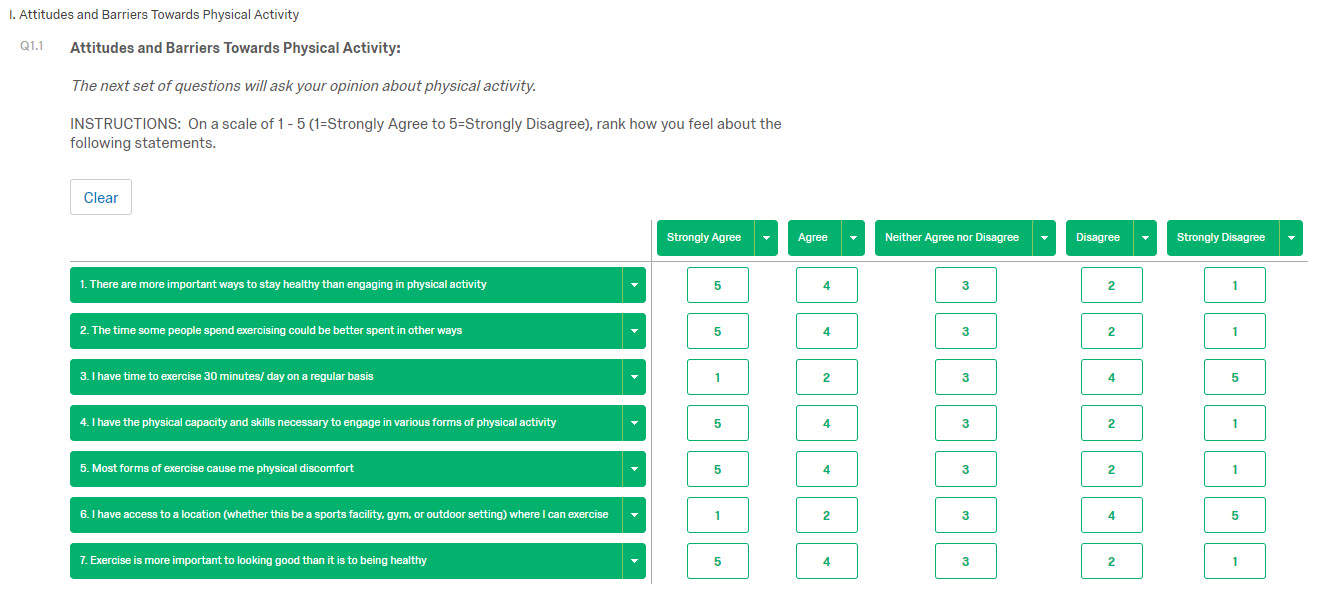The image displays a screenshot of a computer or tablet screen featuring a survey on attitudes and barriers towards physical activity. The background is predominantly white, with text appearing in various shades of gray and black. At the very top, in an extraordinarily small font, the title "Attitudes and Barriers Towards Physical Activity" is presented.

Directly beneath the title, in slightly larger but still very light gray text, is "Question 1.1." Below this, in a darker font, the main heading "Attitudes and Barriers Towards Physical Activity:" is followed by a descriptive subheader in gray and indented, stating, "The next set of questions will ask your opinion about physical activity." 

Following this are instructions, also indented and in the same font style, which read, "On a scale of one to five, from 'Strongly Agree' to 'Strongly Disagree,' rank how you feel about the following statements." Additionally, there is a button that allows users to clear their answers if desired. The scale options are "Strongly Agree," "Agree," "Neither Agree nor Disagree," "Disagree," and "Strongly Disagree," presented in green boxes with clickable buttons beneath each option.

The survey questions listed are:
1. "There are more important ways to stay healthy than engaging in physical activity."
2. "The time some people spend exercising could better be spent in other ways."
3. "I have time to exercise 30 minutes a day on a regular basis."
4. "I have the physical capability to engage in various forms of physical activity."
5. "Most forms of exercise cause me physical discomfort."
6. "I have access to a location, whether it is a sports facility, gym, or similar, where I can exercise."
7. "Exercise is more important for looking good than it is for being healthy."

Each statement has corresponding green boxes for respondents to select their level of agreement.